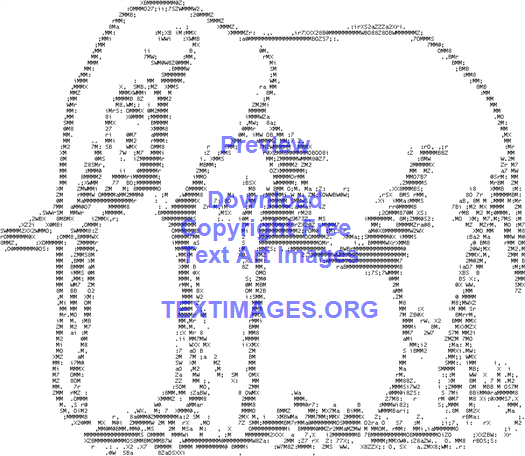The image features a detailed, black and white text art depiction of an elephant in side profile, facing to the left. The elephant's outline and intricate details are constructed from a random assortment of letters, numbers, and symbols, reminiscent of designs produced by old dot matrix printers. Notable characteristics of the elephant include its trunk hanging down almost to the ground, two tusks extending outward, and a visible eye positioned at the front. Additionally, the back of the elephant is adorned with percentages that curve around its short tail. The background of the image is completely blank, enhancing the focus on the text art elephant. Superimposed on the image is blue watermark text that reads, "Preview, Download, Copyright Free, Text Art Images, textimages.org."